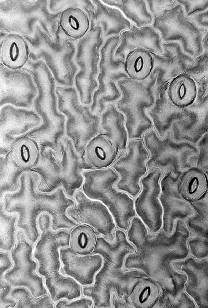This grayscale image resembles a microscopic view, filled with various gray tones ranging from dark to light. It captures an intricate scene akin to observing moisture or bacteria under a microscope, with an array of visual textures and patterns. The depiction includes numerous squiggly, branching shapes bordered by darker gray with lighter gray interiors, interspersed with white and light gray lines. Scattered throughout the image are 10 circular forms, each containing another oblong, oval-shaped outline reminiscent of a cat’s eye pupil. The circles are arranged in a somewhat disconnected pattern, with one in the top left, another slightly above it to the right, and several more scattered diagonally and horizontally across the image, culminating with one near the bottom right and another positioned diagonally upward to the left. The portrait-oriented photograph provides no additional context or labeling, making it unclear whether it is a piece of abstract artwork or a genuine scientific illustration.